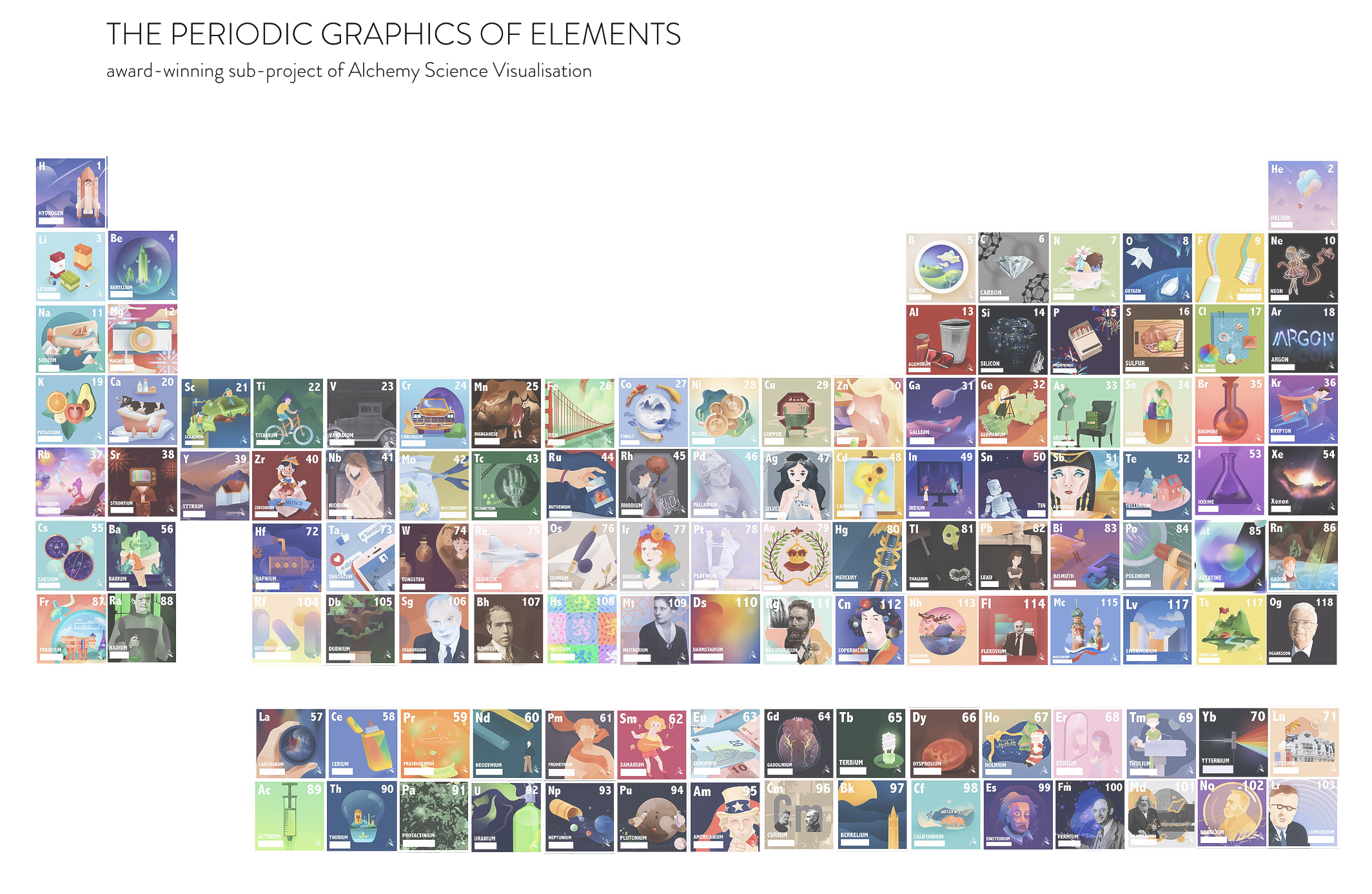This image, entitled "Periodic Graphics of Elements – an award-winning sub-project of alchemy science visualization," features a detailed and colorful representation of the Periodic Table of Elements. The artwork consists of a grid of stamps arranged to form a table-like structure on a white background. Each stamp showcases the atomic symbol in the top left corner and a central picture illustrating various themes such as bridges, people, scientists, fruits, planets, political acts, and scientific tools. The layout exhibits a singular element at both ends of the top row, followed by a series of increasingly longer rows, culminating in sections with rows of up to 10 to 15 elements each. The diverse and vibrant colors of the designs create a visually engaging interpretation of the traditional periodic table.